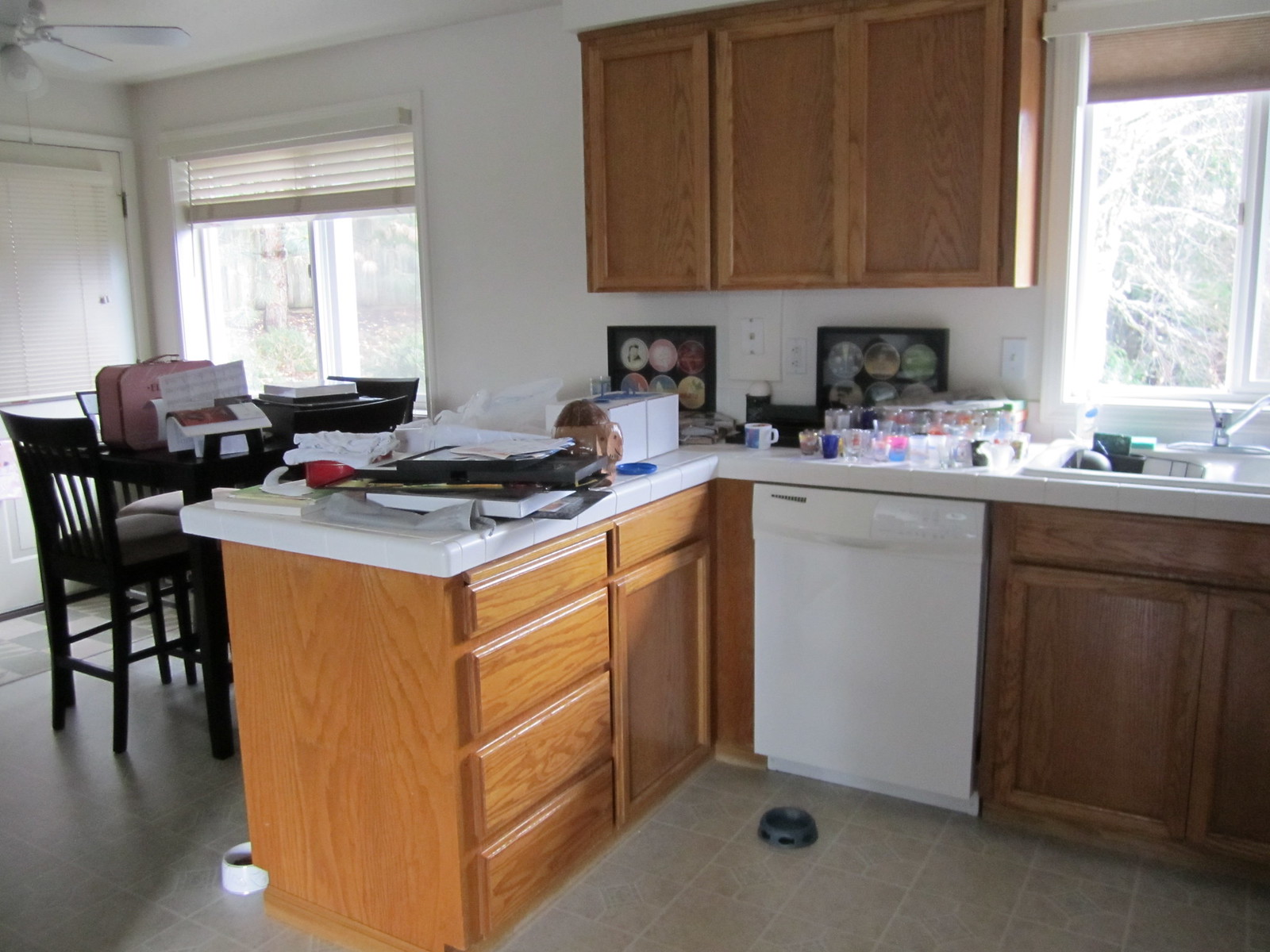This image depicts a cozy kitchen featuring wooden cabinets with a light brown finish and white countertops that resemble marble. Positioned centrally is a white washing machine, flanked by wooden cabinetry. The kitchen includes large windows on both the left and right sides, offering ample natural light, and a view of leafless trees outside. Along the far left wall, a wooden dining table is surrounded by chairs, creating a welcoming dining area. The floor is tiled, and near the dining table, there are two pet bowls for food and water, indicating the presence of a pet in the household. The kitchen's walls are painted white, complementing the bright and airy atmosphere of the space.